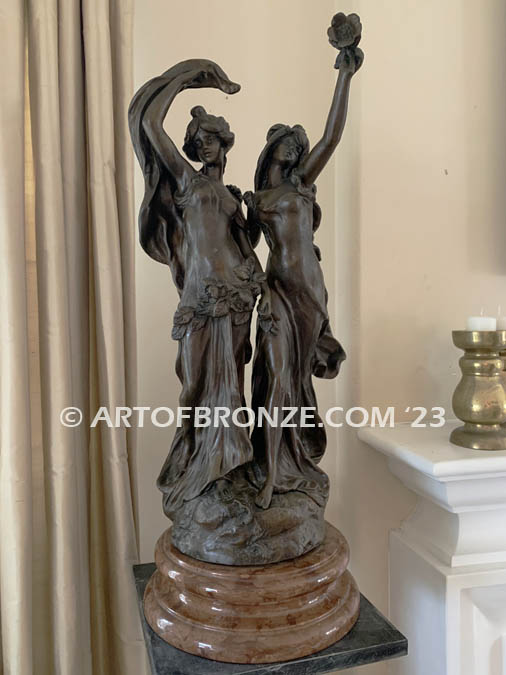This photograph features a bronze statue standing on a multi-layered, marble circular pedestal with a light brown, glossy finish. The statue depicts two elegant, elongated women with their outside arms extended upwards; one raises her right arm, the other her left, evoking a celebratory gesture. Both figures are adorned in off-the-shoulder, flowing dresses that drape down gracefully, detailed with floral or leaf-like embellishments around their waists. Their poses and attire evoke a timeless, classical beauty. The background reveals a softly lit room with beige walls and tan curtains, with a white wooden fireplace mantel visible to one side. Prominently overlaid on the image in white text is a copyright watermark that reads "art2bronx.com23."